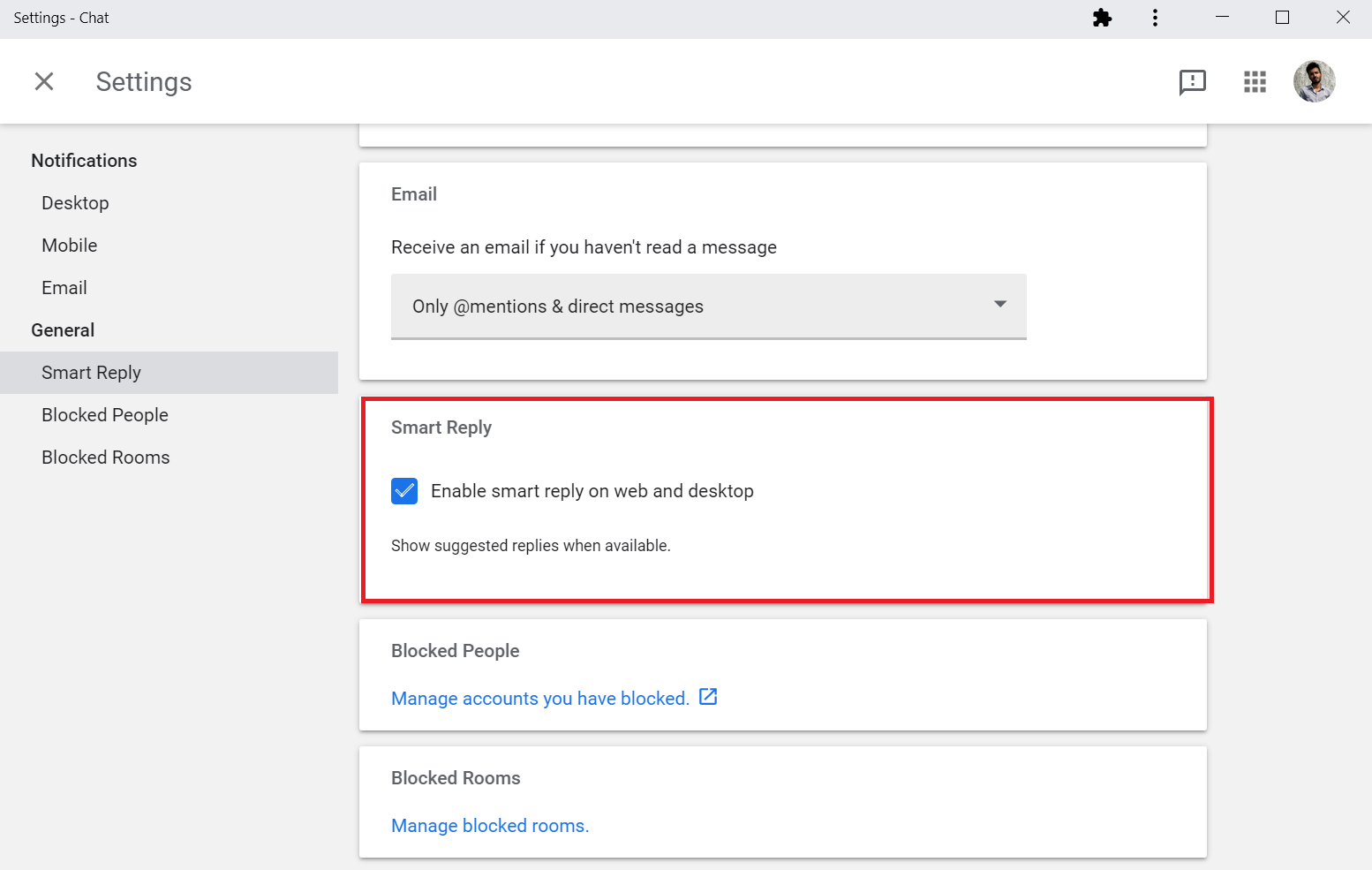The image depicts a chat settings menu on a website. The settings menu is located in the upper left-hand corner of the screen. Directly across from the title "Settings," there's an exclamation mark inside a speech bubble, a keypad icon, and a profile picture.

Below the "Settings" heading, there are several sections. The first section is titled "Notifications" in bold black text, and it covers options for notifications through desktop, mobile, and email. The next main section is "General," also in bold text, where "Smart Reply" is prominently featured.

The "Smart Reply" option is highlighted with a red outline and is currently selected. This section provides an option to enable smart replies on both web and desktop, which suggests automatic replies based on the context of the chat. There's a mention of enabling email if you haven't seen the write-a-message option.

Further down, there are options for managing blocked entities. "Blocked People" allows users to manage accounts they have blocked, and "Blocked Rooms" allows for managing rooms that have been blocked. Both options are marked in blue text, indicating links or actionable buttons.

The overall color scheme is a white and gray background with black text, creating a clear and readable interface. This detailed and organized layout suggests a comprehensive and user-friendly chat settings panel for a web-based platform.